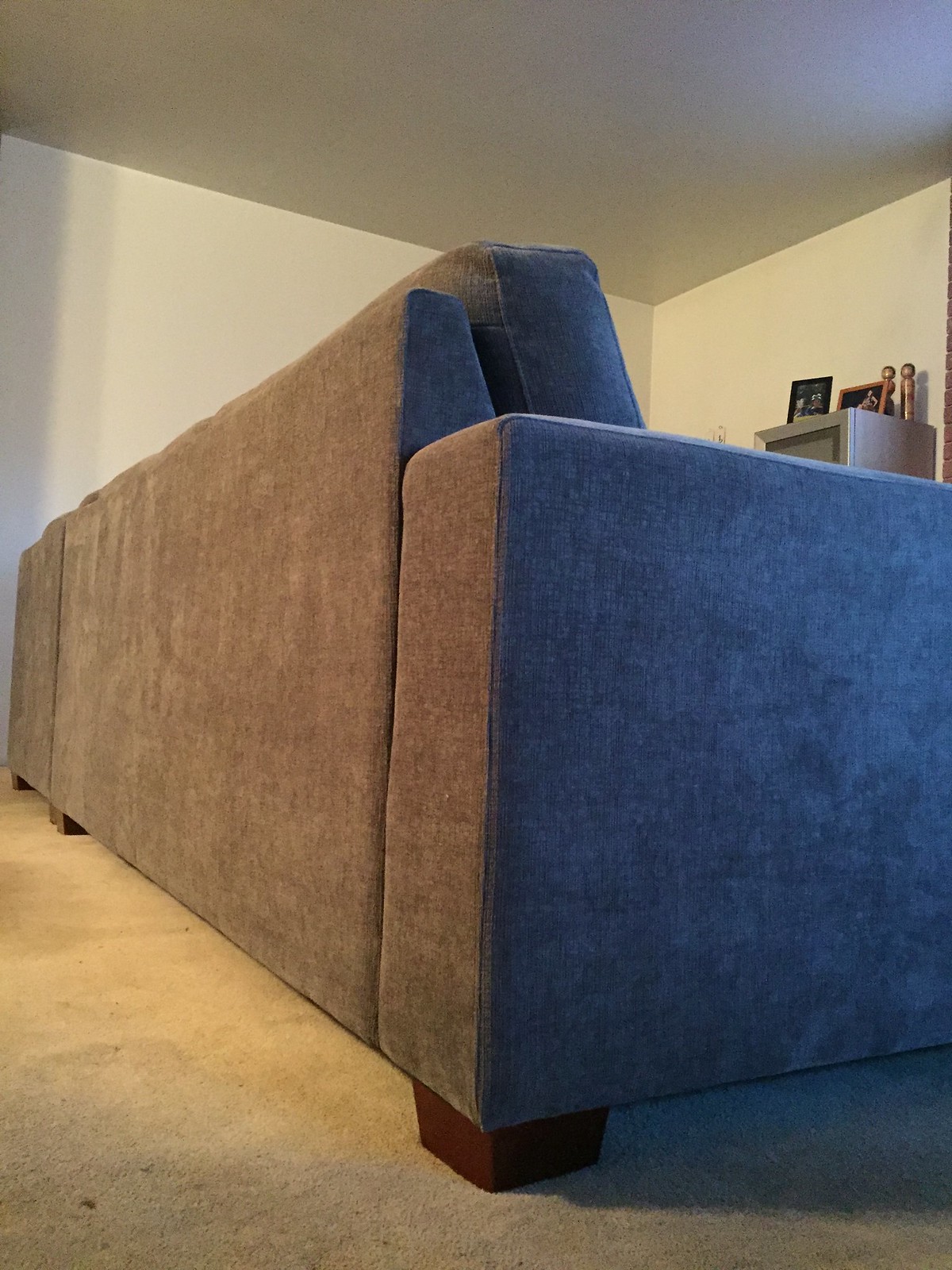In this color photograph of a living room, the focal point is a sleek, modern gray upholstered sofa with short, square wooden legs. Taken from a low angle, the image captures the back and right side of the sofa, which stretches across the left side of the frame and recedes into the distance. The sofa's arm, seamlessly integrated into its side, forms a solid rectangular shape on the right side of the photo. The living room's walls and ceiling are white, contrasting against the beige, wall-to-wall carpeting that shows lighter and darker spots. In the upper right portion of the image, above the line of the sofa, a small television set with photos and assorted items sits on a shelf, adding depth and context to the minimalist setting.